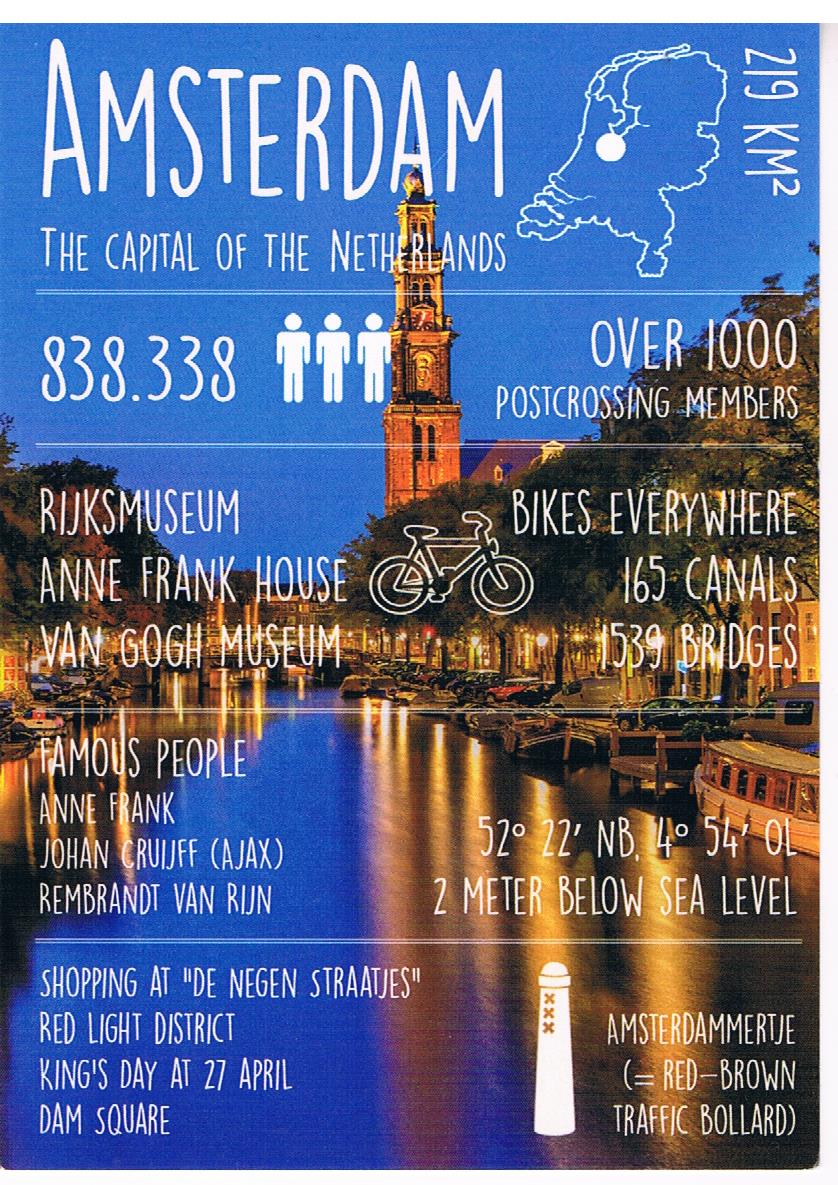The image is a richly detailed information sheet or advertisement showcasing Amsterdam, the capital of the Netherlands. The main photographic background features a picturesque nighttime view of a tree-lined canal bathed in the distinct blue hues of dusk, with the canal's waters reflecting the city's vibrant yellow lights. Prominently placed white text at the top reads "Amsterdam," with a map highlighting the city’s location in the Netherlands. Below, it’s noted as the capital with a population figure of 838,338 and mentions of over 1,000 post-crossing members.

The text overlays highlight notable features of Amsterdam, such as its 165 canals, 1,539 bridges, and the ubiquitous presence of bicycles. There’s a reference to its geographical aspect, being 2 meters below sea level. Cultural and historical landmarks like the Anne Frank House, Rijksmuseum, and Van Gogh Museum are mentioned alongside popular shopping areas like De Negen Straatjes and iconic events such as Kingsday on April 27. Famous personalities associated with the city include Anne Frank, soccer legend Johan Cruyff, and painter Rembrandt van Rijn.

Further details include coordinates (52°22'N, 4°54'E) and several tourist attractions such as the Red Light District and Dam Square. The visual composition includes silhouettes of bicycles and a clock tower, enhancing its informative yet visually appealing presentation.